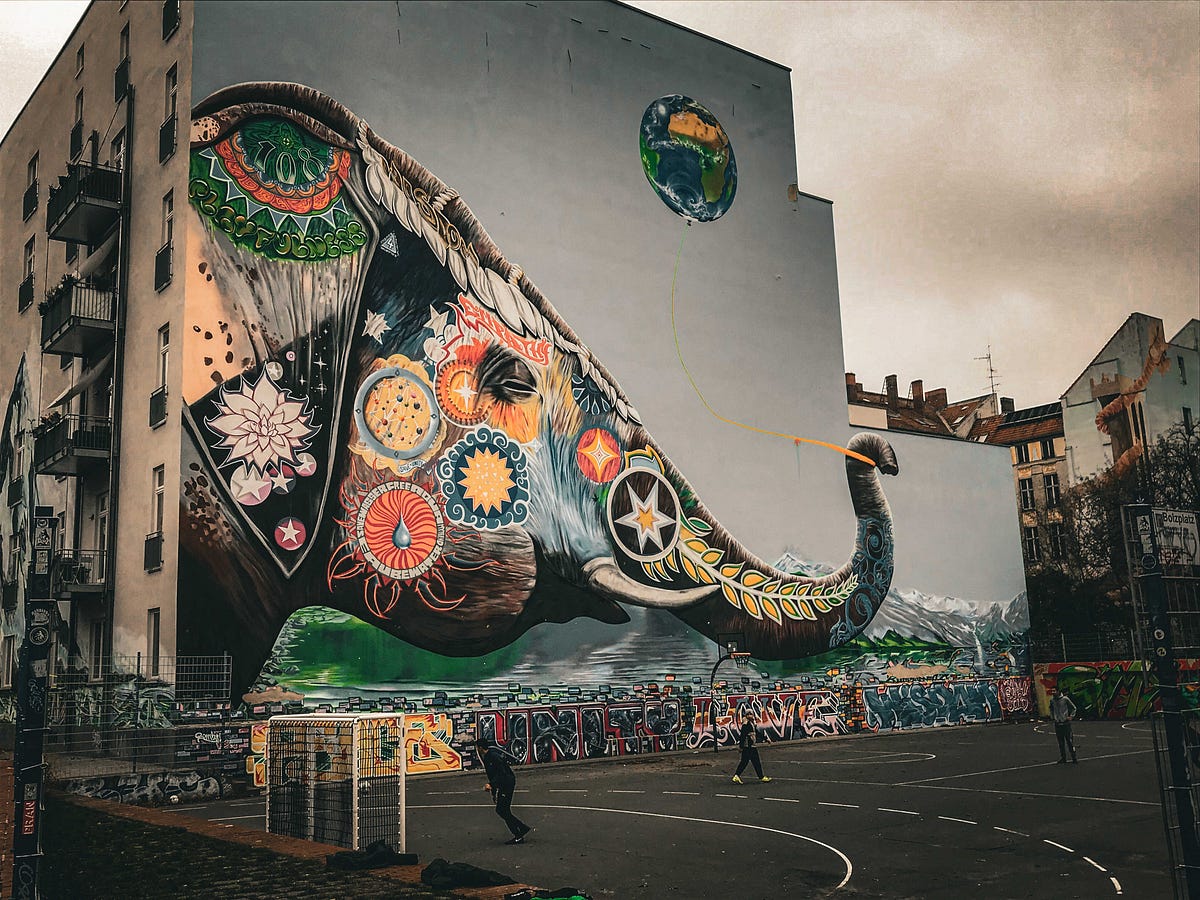This photograph captures the side of a large gray apartment building, prominently featuring an intricate mural of an elephant's head in profile. The elephant's face, adorned with an array of intricate designs including flowers, stars, olive wreath branches, and lotus patterns, is set against a light sky blue background that appears slightly gray due to a filter. The mural also depicts the elephant holding a balloon shaped like the Earth, with a serene scene of a mountaintop and lake further enhancing the background. Below the mural, there are waves and some graffiti. The image is set in an urban area on an overcast day, with three people visible on a black basketball court at the base of the building, engaged in playing either soccer or field hockey. The building also features balconies, adding to its residential feel.